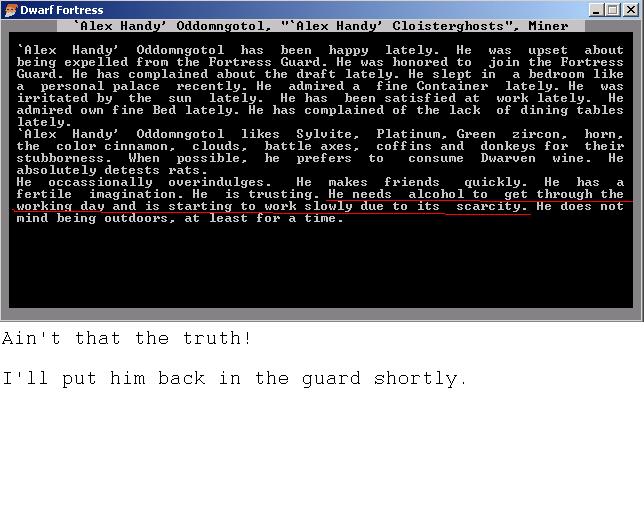This screenshot from the text-based game Dwarf Fortress depicts a profile summary of the character Alex Handy, also known as Ad Amgatal. The top banner in blue reads "Dwarf Fortress," under which the title in gray states, "Alex Handy, Odom Gotol, Alex Handy, Cloyster Ghosts Miner." The main section of the image is a black box filled with gray text detailing Alex Handy's recent sentiments and experiences. The text reveals that Alex has been happy lately but was upset about being expelled from the Fortress Guard despite being honored to join it. He has complained about the draft and the lack of dining tables recently. Alex finds satisfaction in his work and has admired his fine bed and a fine container. He was irritated by the sun and enjoyed sleeping in a bedroom that felt like a personal palace. The text also mentions Alex’s admiration for specific materials and items such as sylvite, platinum, green zircon, horn, the color cinnamon, clouds, battle axes, coffins, and donkeys for their stubbornness. Further character traits reveal that he makes friends quickly, has a fertile imagination, is trusting, relies on alcohol to get through the working day, and is starting to work slowly due to its scarcity. A typewritten note at the bottom of the screen comments, "Ain't that the truth? I'll put him back in the guard shortly."